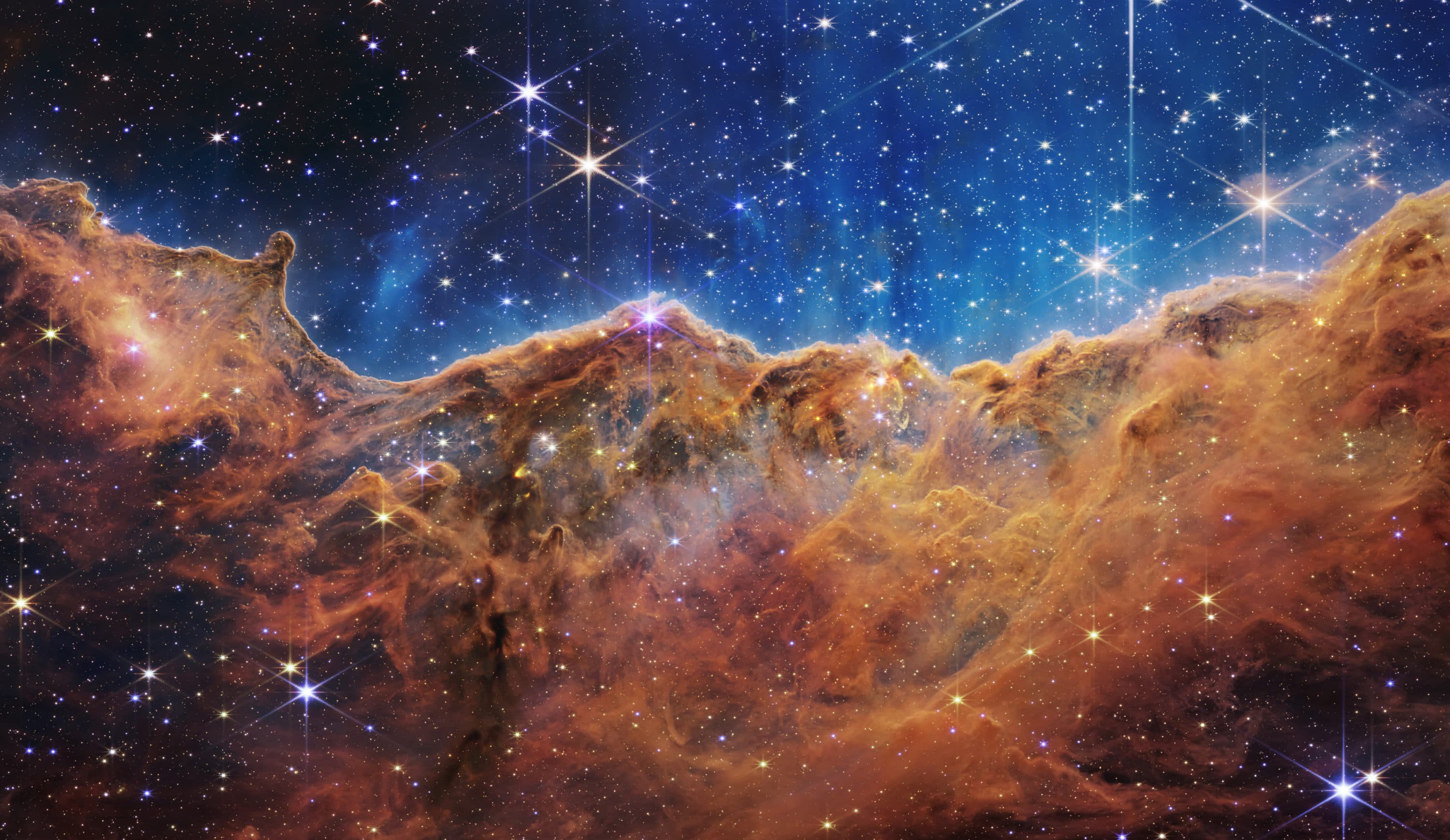A visually stunning computer-generated image of the night sky, likely captured by the Space Web Telescope, showcases a mesmerizing cosmic landscape. The upper portion features a light airy blue atmosphere interspersed with darker patches of black. In the foreground, millions of brilliant white, yellow, and blue stars dot the sky, some with six-pointed rays indicating their brightness. Prominently, three bright stars at the top are either yellow or white, while a few are distinctly blue and have a slight pinkish hue.

In contrast, the bottom half of the image is dominated by a sprawling nebula. This nebulous region is characterized by its dusty, brown coloration, tinged with shades of orange, yellow, and gold. The nebula is a wispy, gaseous formation that stretches horizontally across the canvas and dips slightly towards the center. Despite its smoky, cloud-like appearance, the stars continue to shine through, adding an ethereal quality to the scene. The nebulous clouds also contain some white areas, while the dark and brown hues create a dramatic backdrop against the gleaming stars, encapsulating the grandeur of the cosmos.